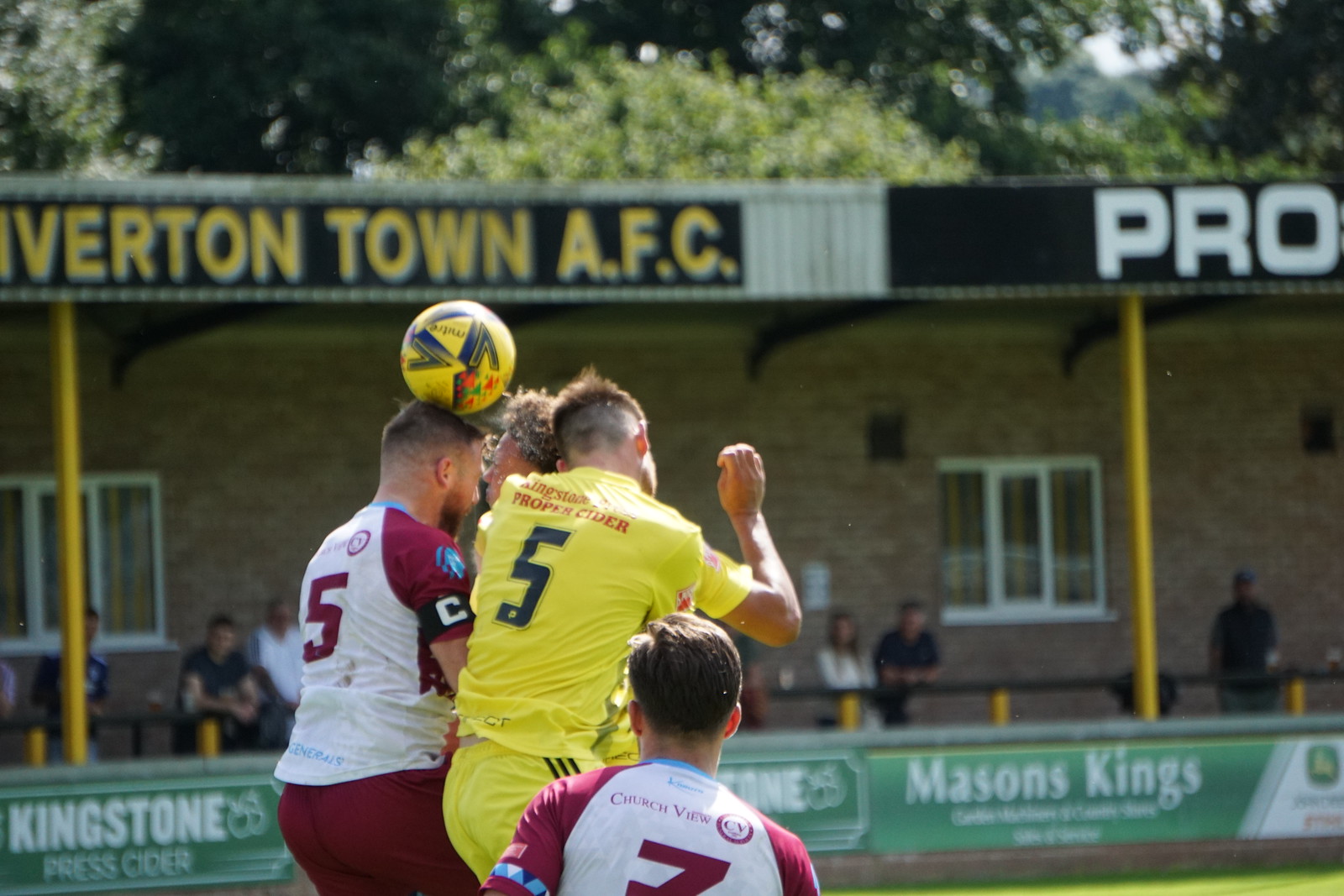The image captures an intense outdoor soccer match, prominently featuring three players at the forefront. Two players from the same team are dressed in burgundy and white uniforms, with the numbers five and seven on their backs. Both players have short brown hair and are viewed from behind. The third player, from the opposing team, is wearing a bright yellow uniform with a blue number five on his back and is also depicted from the back. A yellow and blue soccer ball is being struck in mid-air by one of the burgundy and white-clad players. 

In the background, a modest crowd is observing the action, standing along the rails of a small stadium. The crowd is blurred, as are the green and white advertisements along the bottom of the stands that read "Mason Kings" and "Kingston Press Cider." Above the stands, there is signage with "Everton Town AFC" and "Pro," alongside "Churchview" on the burgundy and white jerseys. Further behind, the scene is framed by lush, green leafy trees, adding a natural contrast to the athletic event.